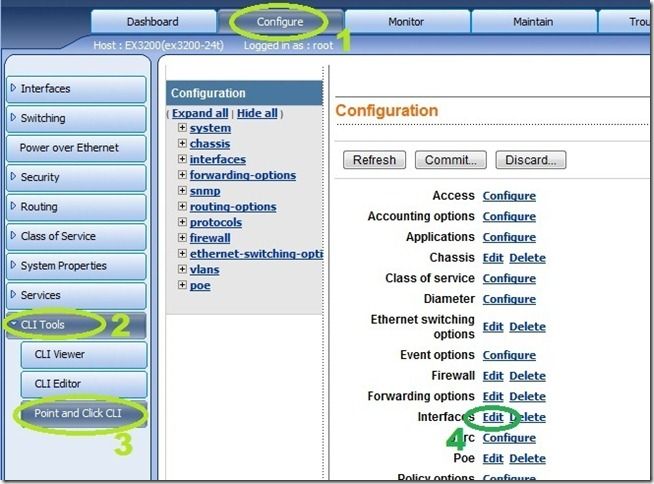The image displays a detailed user interface of a computer software, specifically designed for network management. The central focus of the image is a section with a white background and an orange header labeled "Configuration." Various configuration options are listed here, each highlighted in blue with a gray background, and accompanied by actions such as “Expand All” and “Hide All.”

On the left-hand side, there is a navigation pane featuring multiple sections titled "Interfaces," "Switching," "Power over Ethernet," "Security," "Routing," "Class of Service," "System Properties," and "Services." Additional subsections under "CLI Tools" include "CLI Viewer," "CLI Editor," and "Point and Click CLI," all numbered and circled in lime green. 

In the central dashboard, the word "Configure" is prominently circled in lime green, directing attention to its significance. Many elements, including numbers and text, are presented against a light blue background. A partially visible section that reads "T-R-O-U" indicates part of the word "troubleshooting," though it is cut off.

Overall, the interface is richly detailed, featuring a variety of tools and sections for configuration, monitoring, maintenance, and troubleshooting of network elements.